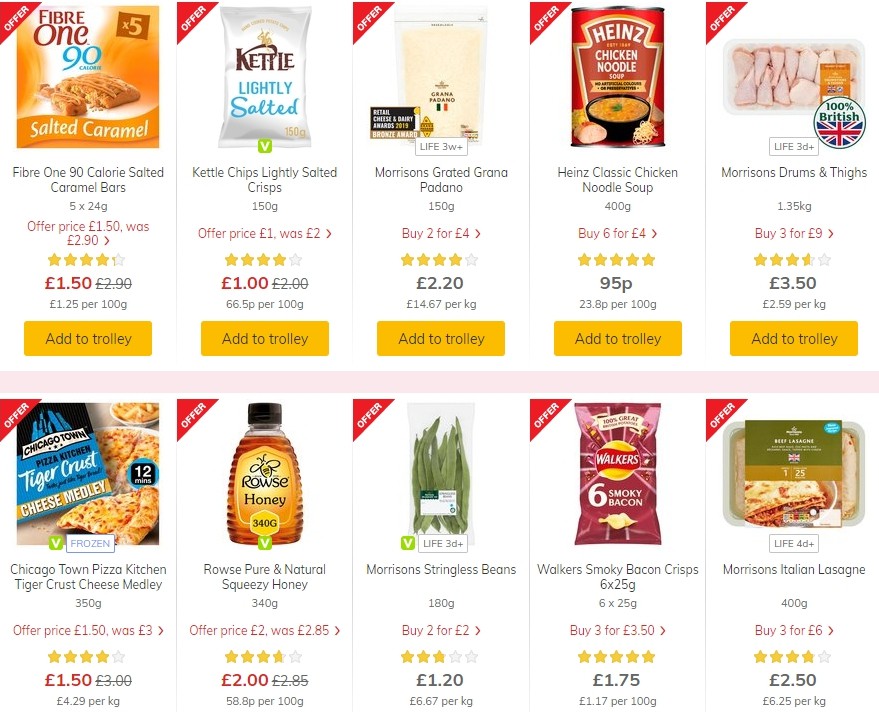Here's the refined and detailed caption:

---

This image is a screenshot of a British e-commerce grocery site. Featured prominently are ten product listings, each marked with a red angled triangle in the upper left corner, labeled "Offer" in white text. Each listing includes an image of the product in its packaging, detailed product name, packaging groupings, gram weight, an offer price, the original price displayed with a strikethrough, a star rating, the current price, and a price per 100 grams. Additionally, there's a yellow "Add to trolley" button below each product.

1. **Fiber One 90 Calorie Salted Caramel Bars**: 
   - Packaging: 5 x 24g 
   - Offer Price: £1.50 (originally £2.90)
   - Rating: Just over 4 stars
   - Price per 100g: £1.25
   - Button: Add to trolley

2. **Kettle Chips**: 
   - No extra specific details provided in text.

3. **Morrison's Grated Grana Padano**: 
   - Notable for being one of the most expensive items.
   - Price: £14.67 per kg

4. **Heinz Classic Chicken Noodle**: 
   - No extra specific details provided in text.

5. **Morrison's Drums and Thighs (Chicken Parts)**: 
   - No extra specific details provided in text.

6. **Tiger Crust Cheese Medley Pizza**: 
   - Looks similar to a quesadilla but is actually a pizza.

7. **Rowse Honey**: 
   - No extra specific details provided in text.

8. **Morrison's String Beans**: 
   - No extra specific details provided in text.

9. **Walker's Smoky Bacon Crisp**: 
   - No extra specific details provided in text.

10. **Morrison's Italian Lasagna**: 
    - Described as one of the most expensive, though precise price details are not given in the text.

Each product's listing is designed to provide comprehensive details to help customers make informed purchasing decisions quickly and easily.